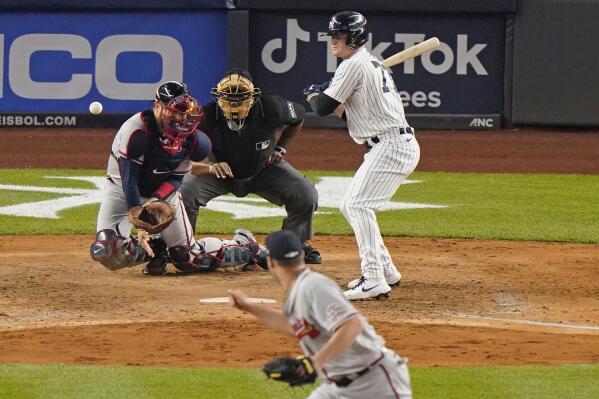This vibrant outdoor landscape image captures a professional baseball game in action. The vantage point suggests the perspective of a spectator standing directly behind the pitcher, who has just hurled the ball towards home plate. The batter, dressed in a classic pinstriped white uniform commonly associated with the New York Yankees, wears a blue helmet and stands in a relaxed pose, seemingly recognizing the pitch as a ball. The catcher and the umpire, positioned right behind the batter, are focused on the trajectory of the ball which is veering off to the left, away from the plate. Surrounding the lush, green, natural turf field with white markings and characteristic dirt patches are ad banners on the padded walls, prominently displaying sponsors "CO", Geico, and TikTok in blue, black, and gray letters, enhancing the professional ambiance of the game.